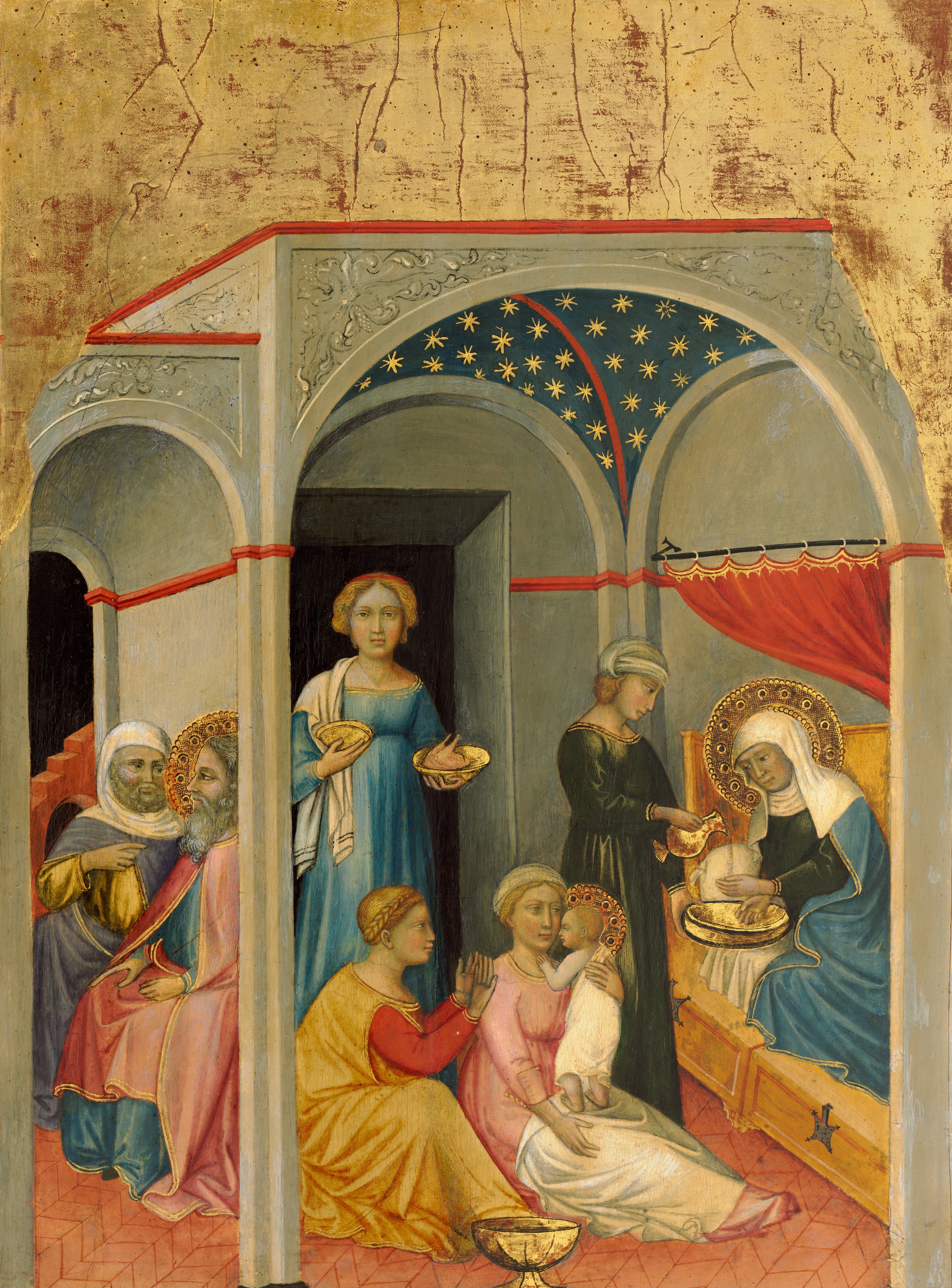This image features a historic artwork that seems to date back around 2,000 years. The artwork is divided into two distinct rooms, their structural elements visible but varying in details. The walls in the background have a brown, tan hue, while the ceiling of the larger room is intricately decorated with a blue sky and yellow stars.

Central to the painting is a woman dressed in a blue gown with a shawl draped around her shoulder, holding a golden plate with what appears to be a Cornish hen. To her left are two men: one in a pink and blue robe with a halo above his head, and the other wearing a head covering and a blue robe. Next to the central woman, a figure clad in a golden robe with red sleeves is seated on the ground alongside another person in a pink robe, who is holding a baby. The baby, also adorned with a halo, is wrapped in a white shroud. 

In the background, a woman is reclined on a yellow, couch-like piece of furniture, with another woman in a dark green dress standing beside her, pouring a liquid over her hands as if in a ritualistic manner. The reclining woman is wearing a white headdress and a blue robe, with a halo around her head too. Although there is great attention to detail, the image lacks any text or explicit context, allowing the viewer to interpret its narrative.